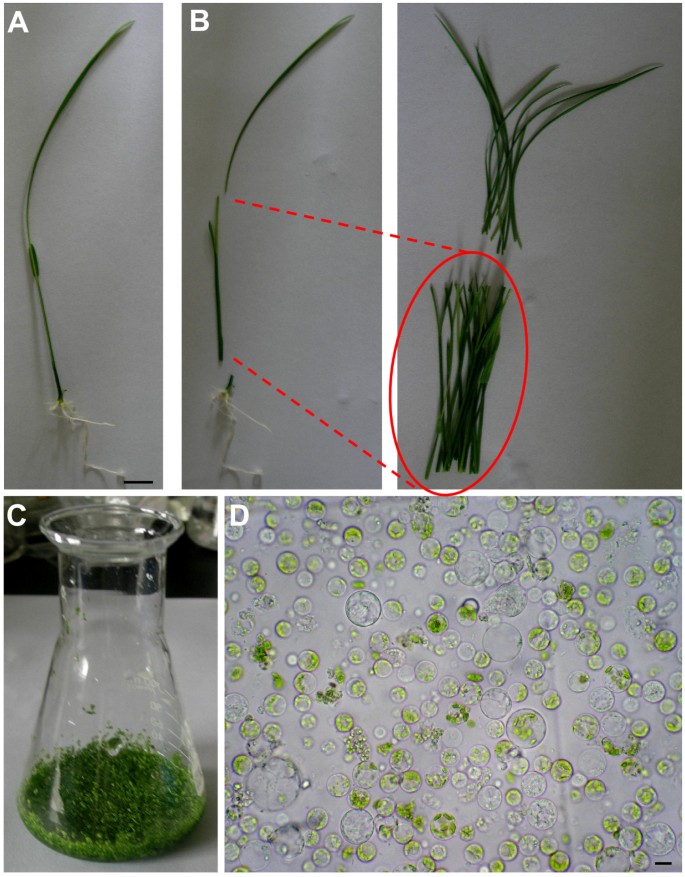The image is a detailed, step-by-step visual guide composed of five labeled photographs. Starting from the top left and moving downward, photograph A displays a tall, green grass-like plant complete with white roots. Photo B, positioned adjacent to A, shows the same plant with the grass part separated from the stalk and the roots cut off, marked by a red outline indicating the cut points. The third photograph, situated to the right of B, enlarges the cut stalks for clarity. In the bottom left corner, image C presents a laboratory beaker filled with a mushy, green substance mixed with liquid, indicative of the plant material being processed. Lastly, photograph D located at the bottom right, provides a detailed view under a microscope, showcasing the green plant cells with various molecules and white bubbles against a gray background, illustrating microscopic examination.